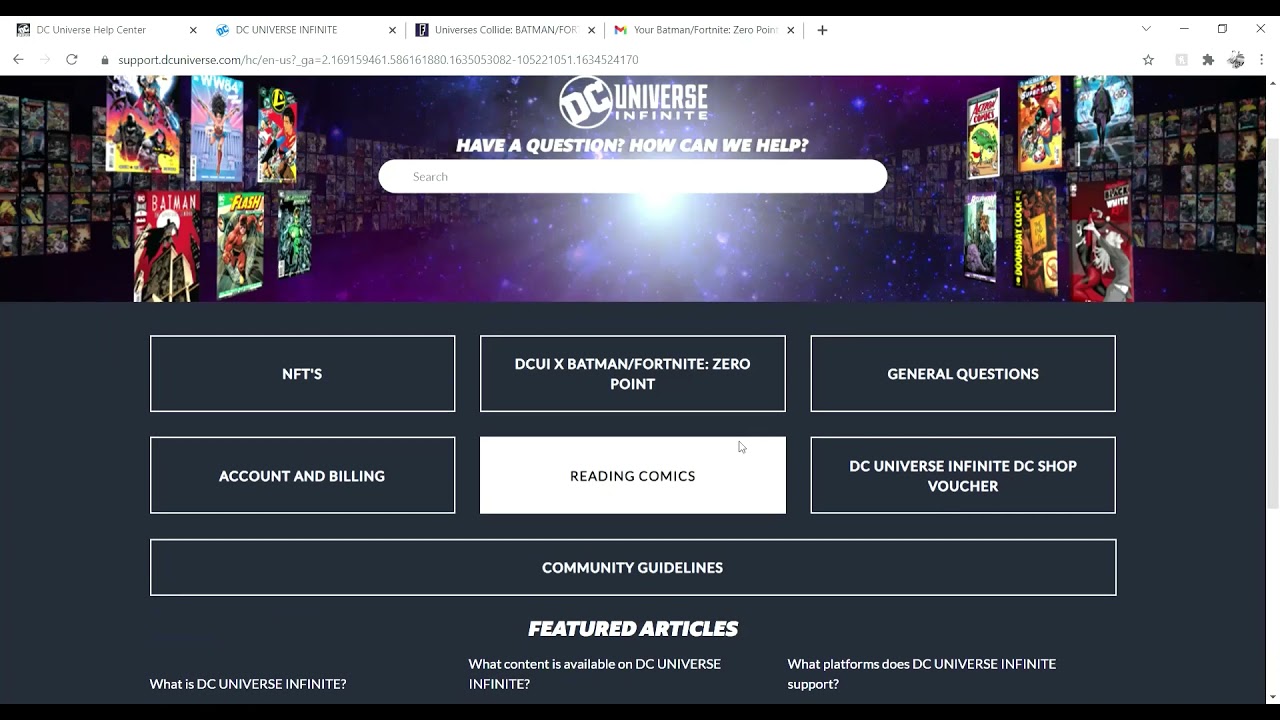Sure! Here is a cleaned-up and detailed caption for the image:

---

The screenshot showcases a webpage viewed in landscape mode on a laptop. The browser interface at the top exhibits several open tabs including, DC Universe Help Center, DC Universe Infinite, Universe Collide Batman, and Email Your Batman/Fortnite Zero. These tabs are situated on a black stripe, followed by white stripes on either side. On the far right is an option to close the browser.

Below the tabs is the URL bar, displaying "support.dcuniverse.com" along with some additional numbers. The main body of the webpage spans the entire width, resembling the interior of a game store with shelves lined with games and CDs.

Dominating the center of the page is a vibrant explosion of a galaxy filled with hues of blue and stars, encapsulating the DC Universe Infinite logo. To the right of this logo, there is a search form for user inquiries titled "Have a question? How can we help?"

On the left side of the screenshot, there are visible images, including at least one Batman and one Flash game. The right side images are less visible. Below, a highlighted box displays "Reading comments" in white text.